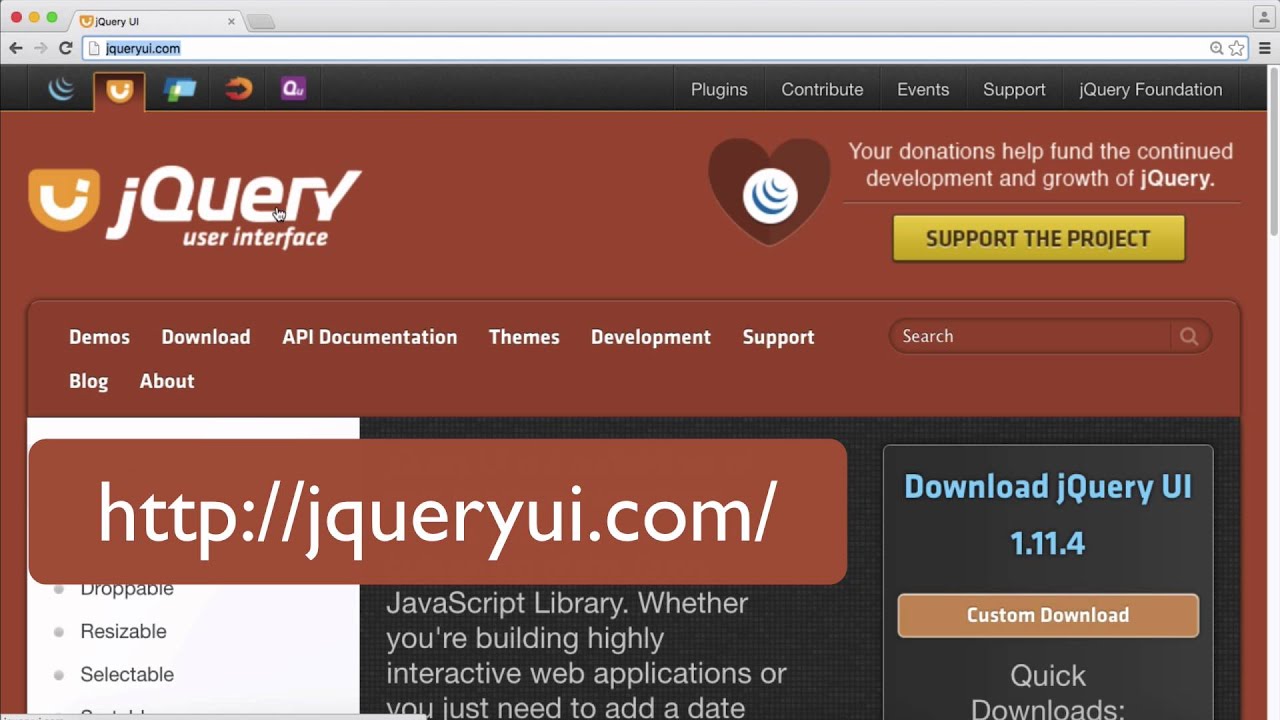The image depicts a webpage from jQuery UI, accessed on an Apple device evidenced by the highlighted URL "http://jqueryui.com" in blue. The open webpage features a black header adorned with glyphs and icons. The header includes navigation links such as "Plugins," "Contributors," "Events," "Support," "jQuery," and "Foundation." An orange-highlighted 'U' on the right side indicates a selected item in a menu, contrasted with a white 'J' representing jQuery User Interface.

Centrally, the background of the page carries a subtle red hue. A notable section on the right emphasizes the importance of donations with the text, "Your donations help fund the continued development and growth of jQuery." Below this message, there’s an orange button labeled "Support the Project," accompanied by a heart icon to its left. The heart possesses a white face inscribed with three curved blue lines. 

Further down, the page contains additional navigation tabs such as "Demos," "Download," "API Documentation," "Themes," "Development," "Support," "Blog," and "About." Adjacent to these tabs, a search box appears on the right. Completing the image, the footer showcases the URL "http://jqueryui.com" in white text against a red backdrop. To the left is a link to "Download jQuery UI 1.11.4" in blue text on a black background, paired with a brown "Custom Download" button.

At the page's center bottom, there's a segment introducing the jQuery library with the statement, "JavaScript library for building highly interactive web applications or adding a date picker," articulated in white text over a black background.